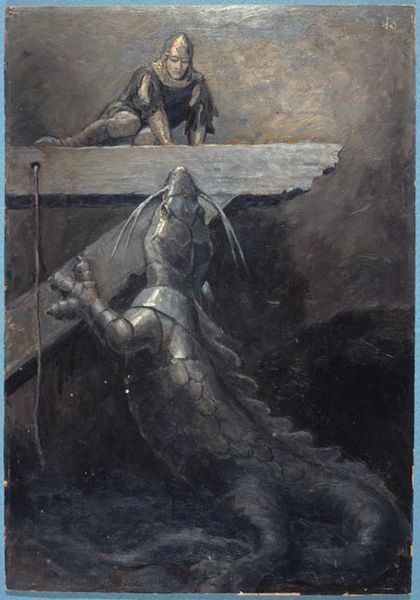This detailed painting, seemingly from medieval times, depicts a dramatic scene of a fearful soldier on a narrow, triangular wooden plank jutting over the water, confronted by a monstrous creature emerging from below. The creature, resembling a large crocodile with the added features of catfish-like whiskers and scales that shine like armor, appears to be lunging towards the soldier. The soldier, clad in chainmail and a conical helmet, embodies the classical medieval look, with his fear clearly evoked as he faces the menacing creature. The overall color palette of silver, gray, and beige gives the scene an almost metallic sheen, emphasizing the armor-like quality of the creature's scales, which mirror the soldier's protective wear. The background and surroundings add depth to the image, depicting an era where mythical sea monsters and armored knights could realistically cross paths.